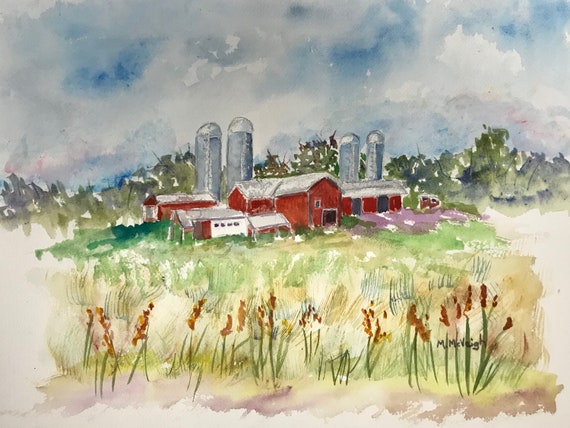In this detailed watercolor painting on a light-colored rectangular canvas, the tranquil rural scene is artfully captured. The painting, with a width twice its height, portrays a serene farm setting rendered in soft, blended hues. Dominating the top section, the sky transitions through light blue, dark gray, and white, with large clouds adding depth and texture.

At the heart of the composition stands a prominent red barn, enhanced with multiple white-framed windows and doorways, as well as a distinctive white garage door. The barn's roof is painted in a light gray, and it is flanked by four tall, cylindrical grain silos, each with dome-shaped tops. Behind the barn stretches a dense tree line, rich with green foliage, contributing to the idyllic backdrop.

In the foreground, the green expanse of a field, likely grass or vegetation, sprawls out with subtle blends of green, brown, and white. Adding to the charm, the bottom part of the painting features slender, tall leaves with brown tips, and yellow-brown flowers contributing pops of color near the ground. Notably, the meticulous details extend to a signature found in the lower right corner, inscribed with the name “M. McVeigh,” affirming the artist’s identity and adding a personal touch to this picturesque farm scene.